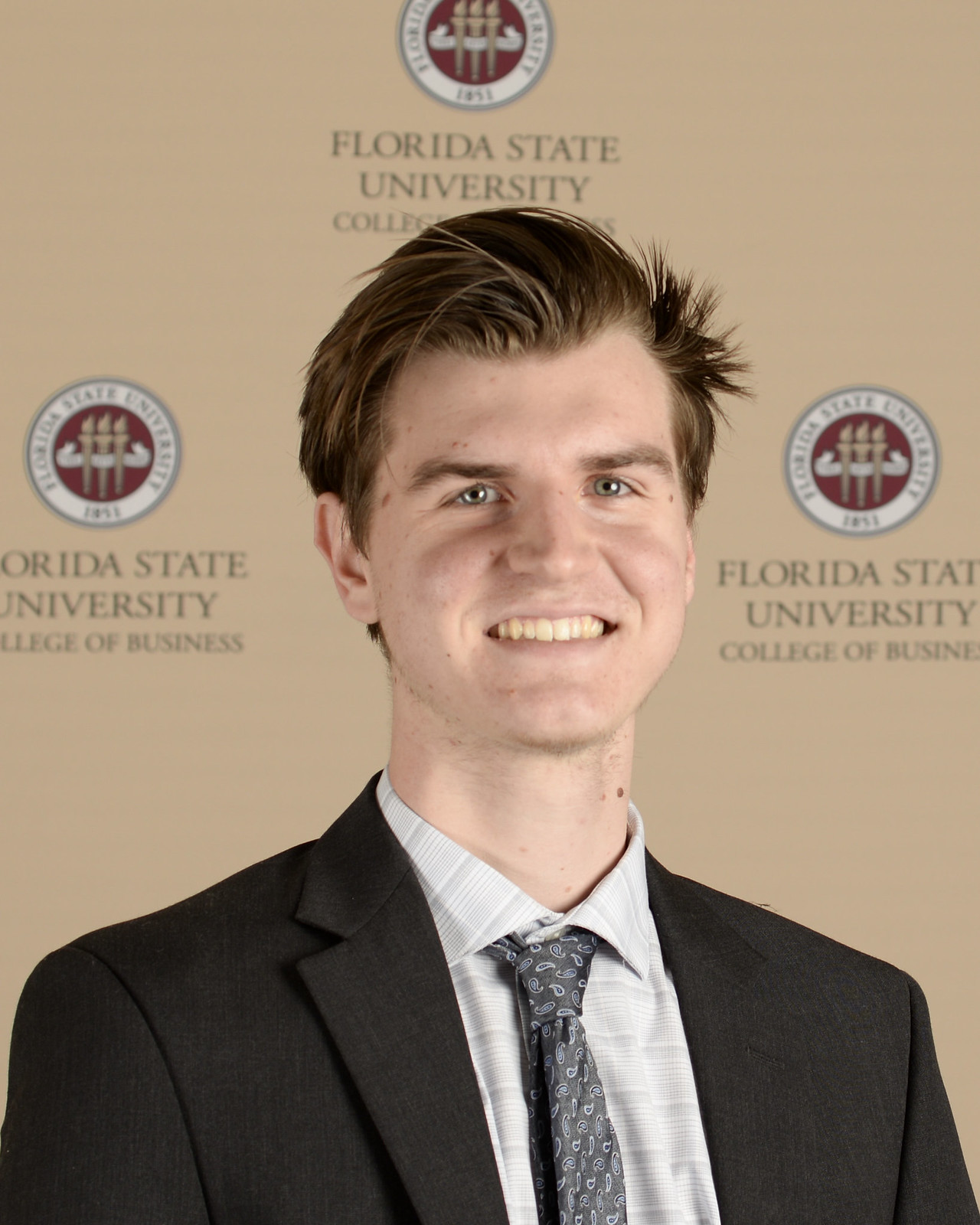This photograph features a poised man standing in front of a beige, almost peach-colored wall with the Florida State University College of Business emblem and name repeated three times: one above his head and one on either side. He has short, reddish-brown hair, fair skin, thick eyebrows, and hazel or blue eyes. He is dressed in a dark gray blazer with a light blue button-down shirt featuring a subtle square pattern, and a dark blue paisley tie. The subject, who presents as male, is smiling warmly, suggesting a formal, celebratory occasion such as graduation.